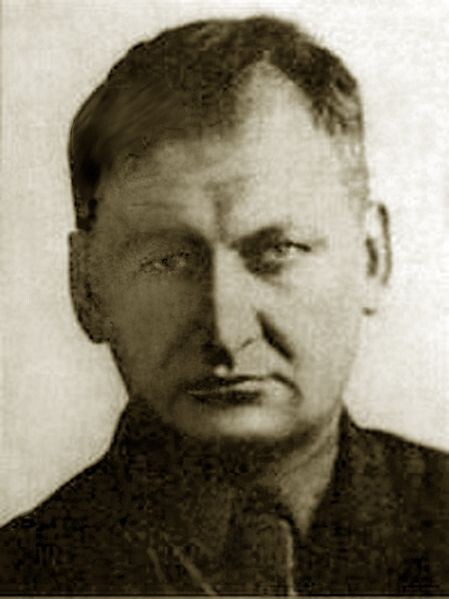The image depicts a middle-aged, Western-origin man set against a pale grey background. He has short brown hair neatly parted at the side and cut above his ears. His face is etched with the signs of age, including noticeable wrinkles on his forehead and two prominent lines stretching from the sides of his nose towards the corners of his closed mouth. He has a long, straight nose and slightly asymmetrical eyebrows, with one lower than the other. His sad, withdrawn eyes, matched by his downturned mouth, convey a sense of hopelessness. He wears a dark brown suit jacket over a grey collared shirt, paired with a brown tie. The image is in sepia tone, adding an aged appearance to the photograph. Despite facing the camera, the man’s eyes seem to stare into the distance, giving an impression of deep contemplation or sorrow. The background shows some shading, with the right side of the image being slightly brighter.